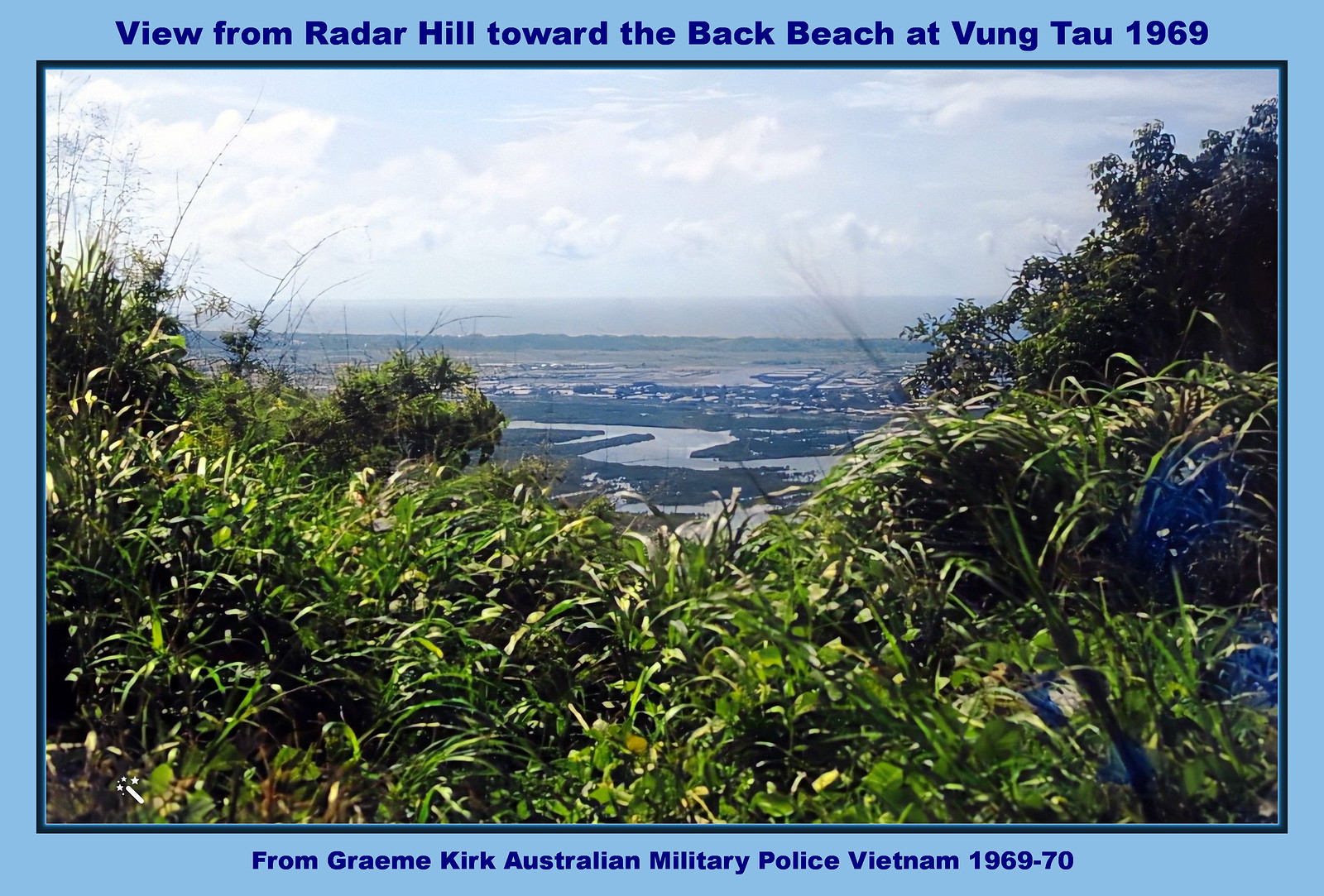This is an outdoor photograph set against a light blue background with dark blue text above and below it. The top of the image reads, "View from Radar Hill toward the back beach at Vung Tau 1969," and the bottom text states, "From Graham Kirk, Australian Military Police, Vietnam 1969-70." The photo captures a scenic overlook from Radar Hill, featuring a lush, green landscape covered with tall grass, short vegetation, and clusters of small trees. In the forefront, there is tall, lush grass, and on the right-hand corner, three distinct purple flowers. The terrain includes a serpentine river winding through the greenery, leading to distant mountains and what appears to be a city or buildings. The day is beautifully captured with a blue sky dotted with white clouds, adding depth to the vibrant outdoor scene. The image invokes the serene yet detailed landscape of Vung Tau during the late 1960s.